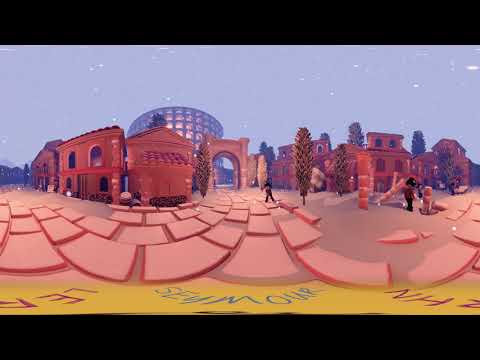The image is a panoramic fisheye illustration created by combining two similar images, enhanced with special filters to produce a cartoonish, claymation effect. It is presented in landscape orientation, framed by horizontal black strips at the top and bottom. The scene features several rose-colored stucco buildings with tile roofs, including a two-story structure and a large circular building with high glass walls that dominate the center. In the foreground, there is a curved courtyard paved with large, pink, rectangular tiles. Scattered around the buildings are several tall cypress trees, adding to the scenery's depth. There are also a couple of indistinguishable objects and two people, who appear cartoonish from this distance. At the bottom, there is a yellow strip containing red and blue lettering, likely filter information, but it is mostly illegible, with notable letters being "LEP" and "C more." The image exudes a whimsical, almost surreal atmosphere, blurring the line between reality and illustration.